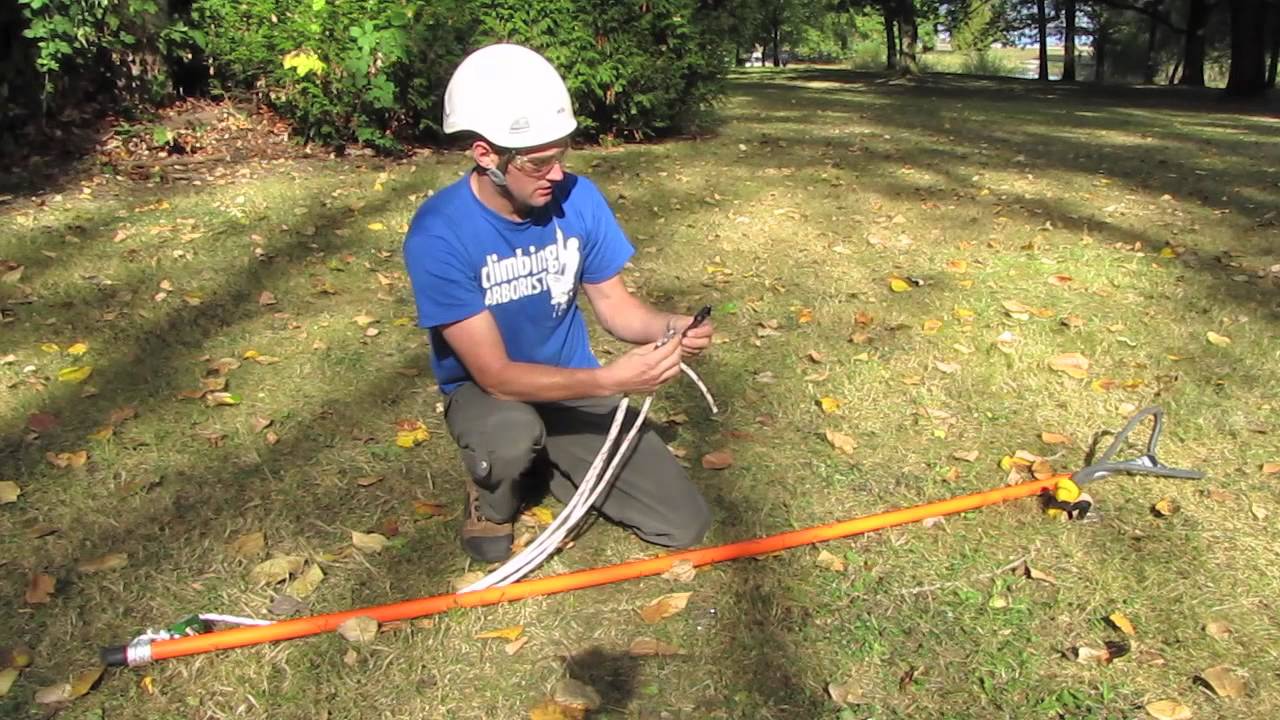In the image, a man is depicted crouching down in a grassy area that suggests a forested setting or a well-maintained backyard. Fallen leaves on the not-so-green grass signal it might be fall. The man is intently working on a pole saw, a long tool typically used for cutting high branches. The base of this tool is a distinct orange and red color, and it has some white wires emerging from it. He’s adjusting a rope connected to the tool between his hands. 

The man is dressed for safety, wearing a white helmet and clear safety goggles. He has on a blue shirt with white text stating "Climbing Arborist," which also features a silhouette of a person climbing. Complementing his outfit are dark gray pants and sturdy brown work boots. The surroundings include a few trees and some shrubbery in the background, with tree shadows cast on the ground, suggesting that the scene takes place in daylight.